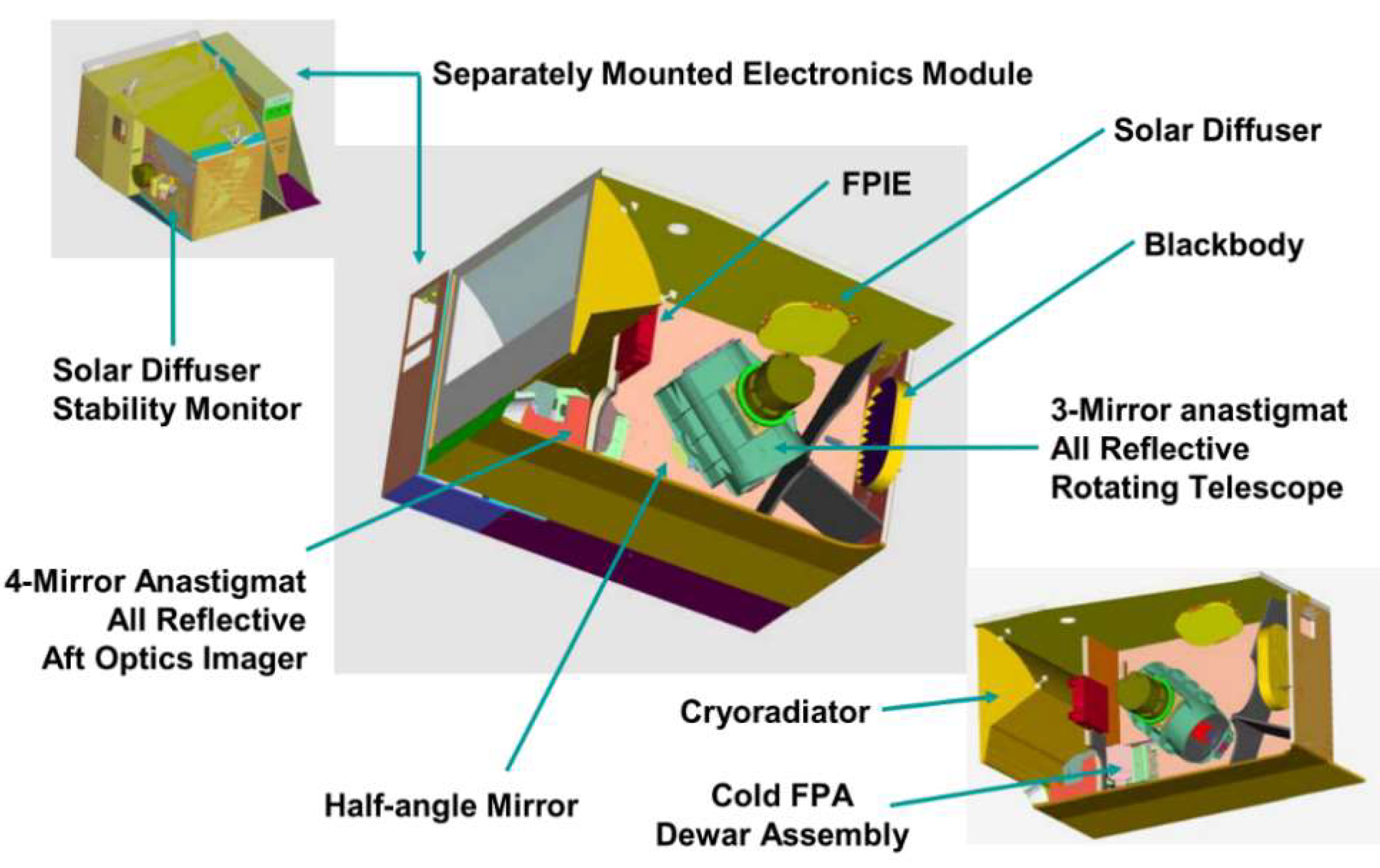The image is a detailed diagram highlighting various components of an electronic device, displayed through three distinct illustrations against a white background. The illustrations are arranged with a smaller one in the top left corner, a larger one in the center, and another smaller one in the bottom right corner, all connected and set against a subtle gray backdrop. The device is encased in green housing with colorful internal components, including purple interiors and variously colored parts.

Key parts are identified with teal arrows and labels, such as a "solar diffuser stability monitor" connected to the green housing, a "four-mirror anastigmat all reflective AFT optics imager" linked to a red component in the upper left image, and a "half angled mirror" highlighted in the center image. Other critical components include the "black body" on the right side of the green box, a "three-mirror anastigmat all reflective rotating telescope," and a "cryo-radiator cold FPA Dewar assembly," depicted from different angles in the central and lower right images.

The middle and largest image shows the internal layout more clearly, spotlighting parts like the "FPIE," another solar diffuser, and the intricate assembly of mirrors and optical elements. The illustrations, though not realistically detailed, provide a clear understanding of the spatial arrangement and functional connections of the device's components, making it evident that these are hand-drawn depictions rather than actual photographs.